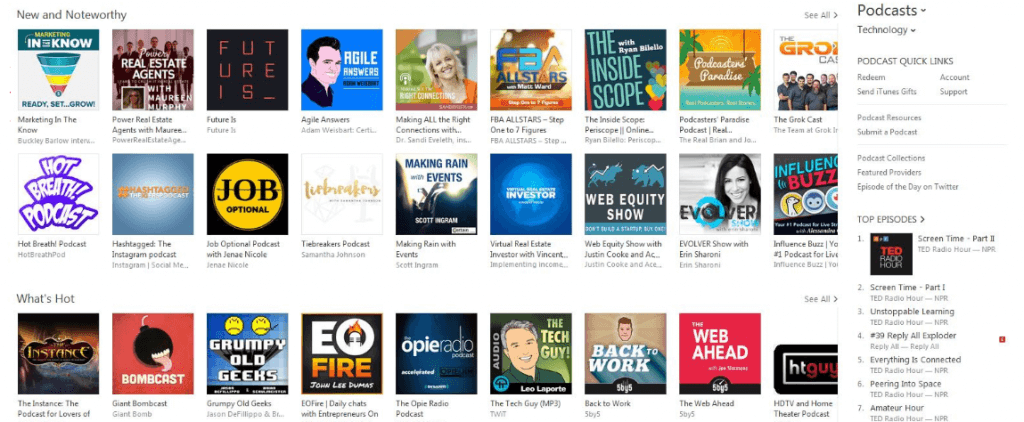This image is a horizontal screenshot of a podcast directory page, prominently featuring icons and titles of various podcasts. A vertical scroll bar on the right side reads "Podcasts under Technology, Podcast Quick Links," while at the bottom of this section is a label for "Top Episodes." The number one top episode listed is "Screen Time Part 2" from TED Radio Hour, identified by a small icon.

The main section of the screenshot comprises three horizontal rows of podcast icons, each row containing nine podcasts, although the ninth podcast is partially obscured by the vertical scroll bar. 

**Top Row:**
1. Marketing in the Know
2. Power Real Estate Agents
3. Future Is
4. Agile Answers
5. Making All the Right Connections
6. FBA All-Stars
7. The Inside Scope
8. Podcasters Paradise Podcast
9. The Grok Cast

**Second Row:**
1. Hot Breath Podcast
2. Hashtagged
3. Job Optional Podcast
4. Tie Breakers Podcast
5. Making Rain with Events
6. Virtual Real Estate
7. Web Equity
8. Evolver
9. Influence Buzz

**Third Row (Under "What's Hot"):**
1. The Instance
2. Giant Bomb Cast
3. Grumpy Old Geeks
4. EO Fire
5. The Opie Radio
6. The Tech Guy
7. Back to Work
8. The Web Ahead
9. HTTV

Each podcast is represented by a square picture above the text title, and the icons above the text labels are rainbow-colored.